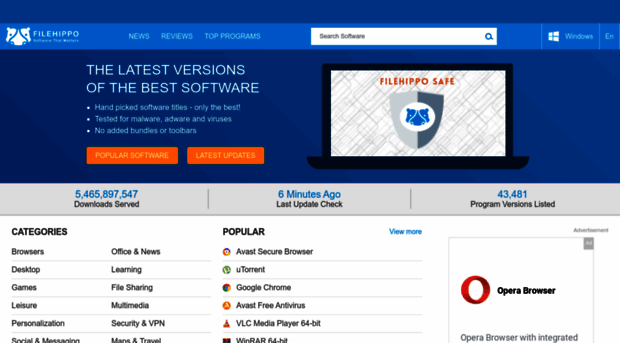Screenshot Description:

The screenshot displays a clean white background featuring the latest versions of popular software. A laptop is prominently shown with two orange rectangles highlighting certain areas. At the top of the screen, there is a search bar with a blue magnifying glass icon and the text "Windows EN" positioned nearby.

The header includes navigation options: "FILEHIPPO," "News," "Reviews," "Top Programs." The site boasts an impressive statistic of "5,465,897,547 downloads served" highlighted in a prominent position. 

Additionally, there is a timestamp indicating that the last update check was performed "six minutes ago." Below this information, the site lists "43,481 program versions" available for users.

The categories for software are listed methodically, including Browsers, Desktop, Games, Leisure, Personalization, Office, News, Learning, File Sharing, Multimedia, Security, and VPN.